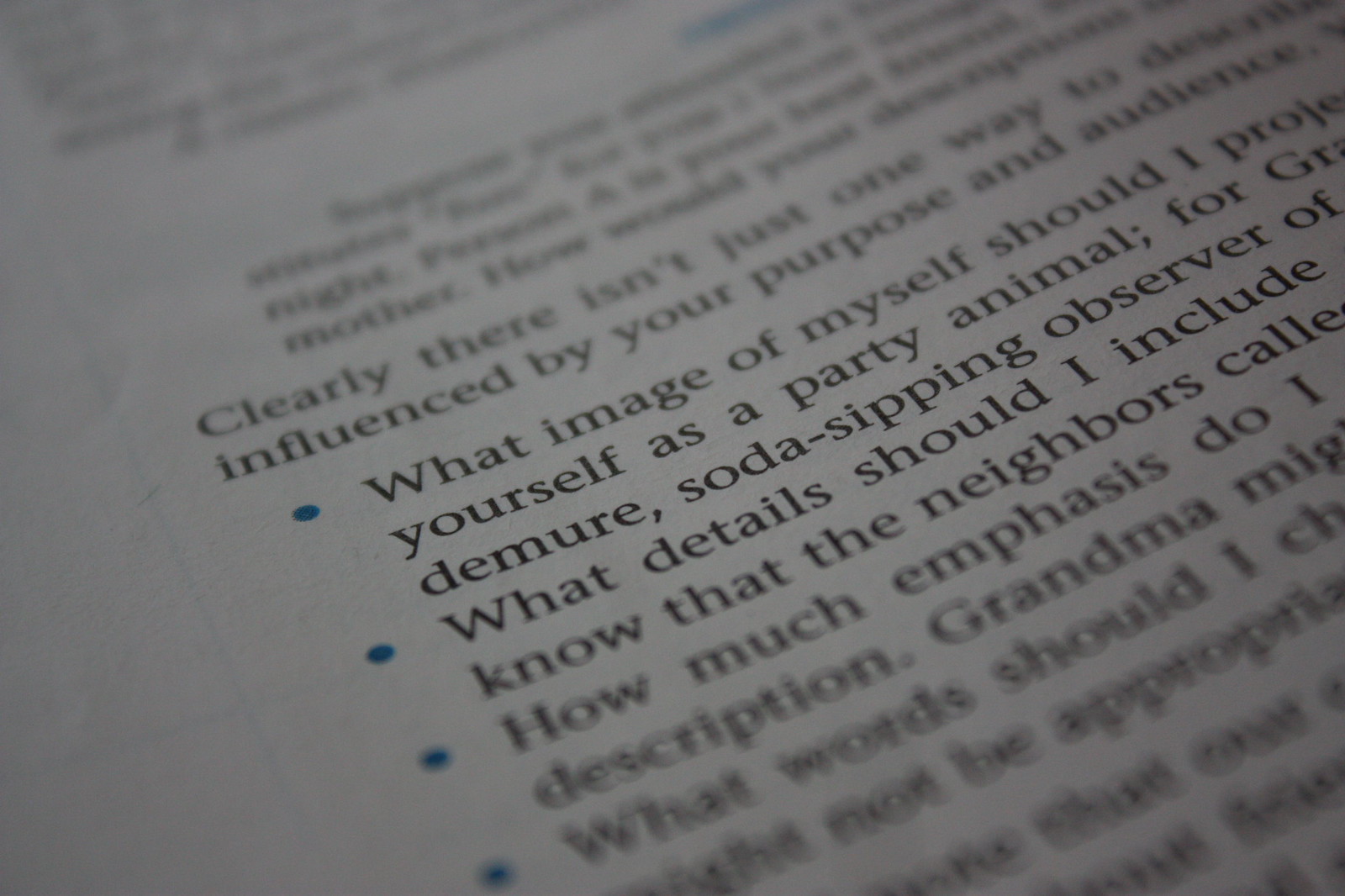This image features a photograph of a book or a page from a book, where most of the text is black on a gray background—possibly due to the lighting. The text includes several sections, with some portions blurred and others clearly visible. Bullet points, indicated by deep blue dots, enumerate various points from top to bottom, with four points in total. The legible parts suggest a focus on topics like personality, influence, purpose, and audience, possibly discussing self-improvement or self-perception, as inferred from phrases like "influence by a purpose and audience" and hints about different personal images.